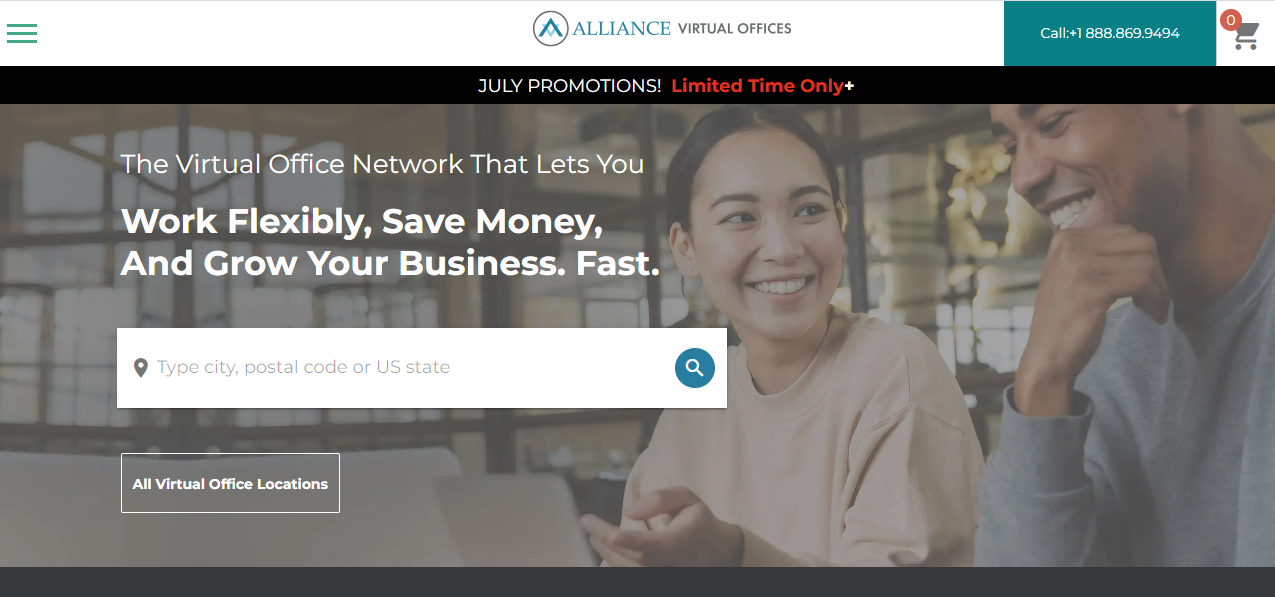The image showcases the homepage of Alliance Virtual Offices. On the left side, the design begins with three vertically stacked green lines. Below this, the background is primarily white. On the right side of the image, there is a prompt to "Call 1-888-869-9494" set above a teal background with white text. Adjacent to the teal section, there is a white background with a shopping cart icon, featuring a red circle with a '0' at its top right corner.

Beneath this section, a black band displays the text "July Promotions" in white and "limited time only" in red. Following this is a photograph of a smiling woman and man, both seated at a table and engaged in conversation. The woman is Asian and the man is Black. Overlaid on the photograph is a slogan in white font: "The virtual office network that lets you work flexibly, save money, and grow your business fast." 

Below this text lies a search bar carrying the placeholder text "type city, postal code, or U.S. state," written in gray on a white background. The search button beside it is a teal circle featuring a magnifying glass icon. Further down, there are buttons to view all virtual office locations. The entire layout is enclosed at the bottom with another black band. The predominant colors in the image are red, gray, black, and teal.